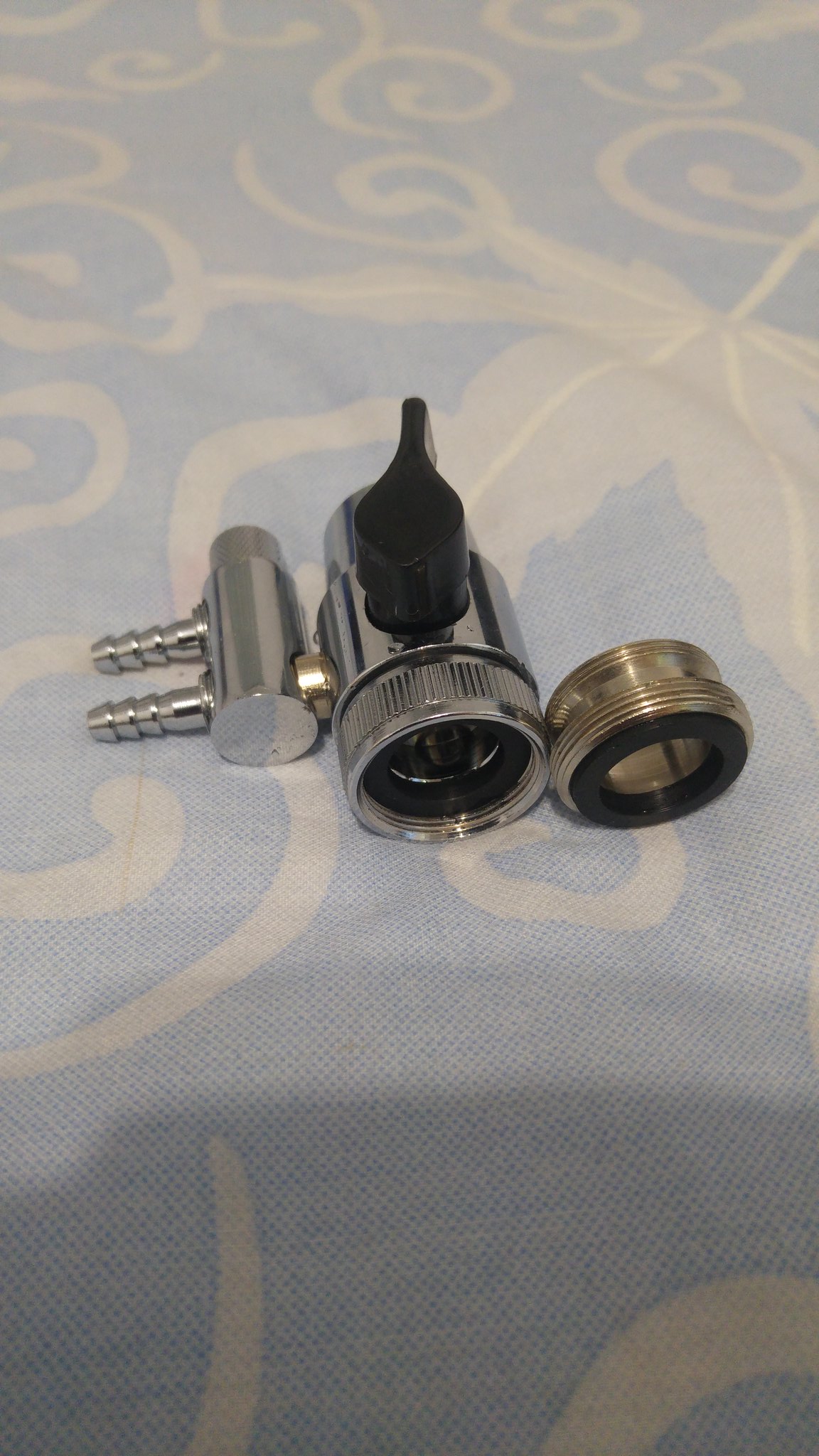The photograph, taken from above, features a detailed piece of hardware resting on a blue tablecloth adorned with curly, ornate white designs. Dominating the center of the image is a compact, silver cylindrical device that resembles a miniature camera lens. This lens faces downward due to the angle of the shot. On the left side of the main cylinder, there's a silver tube about two inches long, equipped with two horizontal screws that suggest it can attach to other components. Atop this central device sits a round black plastic knob with a stick extending backward, which appears to control the opening or closing of access within the tube. On the right side of the apparatus, a small gold item, possibly the end of a mini camera lens, aligns perfectly as if it can be screwed into the central cylinder. The interconnected metal pieces, displaying a blend of silver and gold, highlight a complex, tightly integrated piece of hardware.